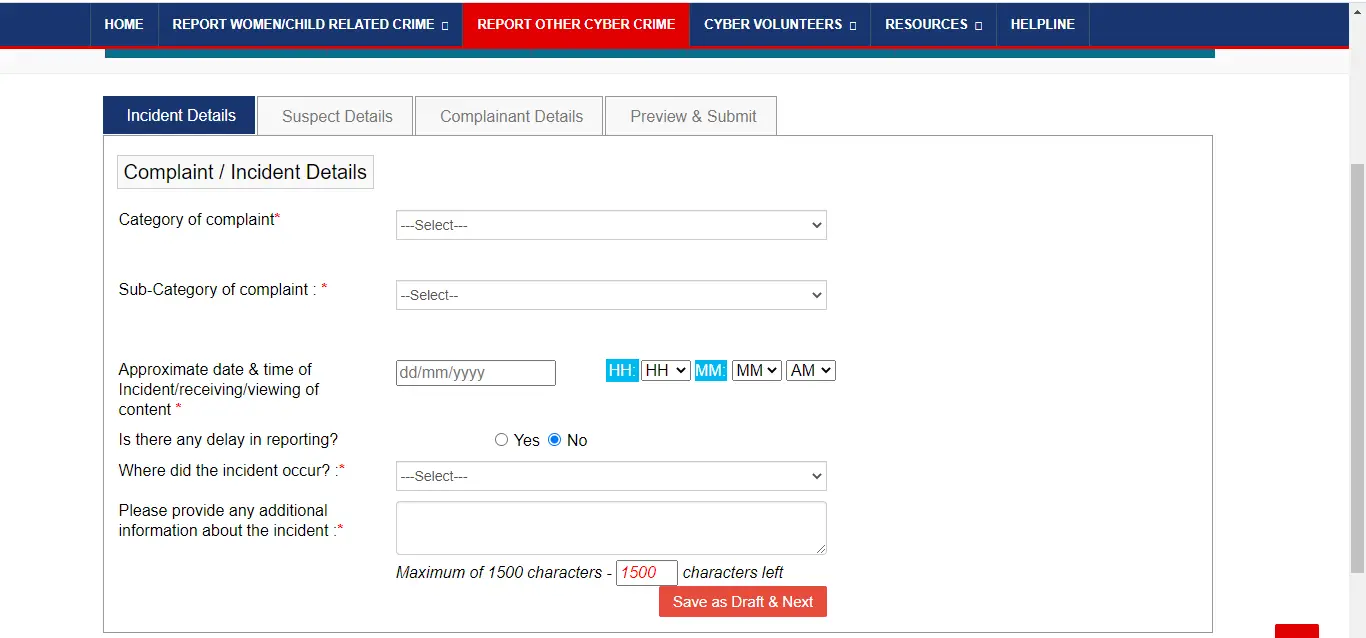The image is a detailed screenshot of a website interface designed for reporting various types of crimes. At the top of the webpage, there are multiple navigational tabs labeled sequentially as: "Home," "Report Women/Child Related Crime," "Report Other Cybercrime," "Cyber Volunteers," "Resources," and "Helpline." The currently active tab, highlighted in red, is "Report Other Cybercrime." 

Within this active tab, the user is in the "Incident Details" section. Here, there are several interactive fields and prompts for the user to fill out. The section header reads "Complaint/Incident Details." Below this, there is an empty drop-down box for selecting the "Category of Complaint," followed by another drop-down box for the "Subcategory of Complaint." There are further prompts for specifying the "Approximate Date and Time of Incident" and for noting if there is any delay in reporting the incident ("Is There Any Delay in Reporting?"). Additional fields include "Where Did the Incident Occur?" and a larger text box labeled "Please Provide Any Additional Information About the Incident" for more comprehensive details.